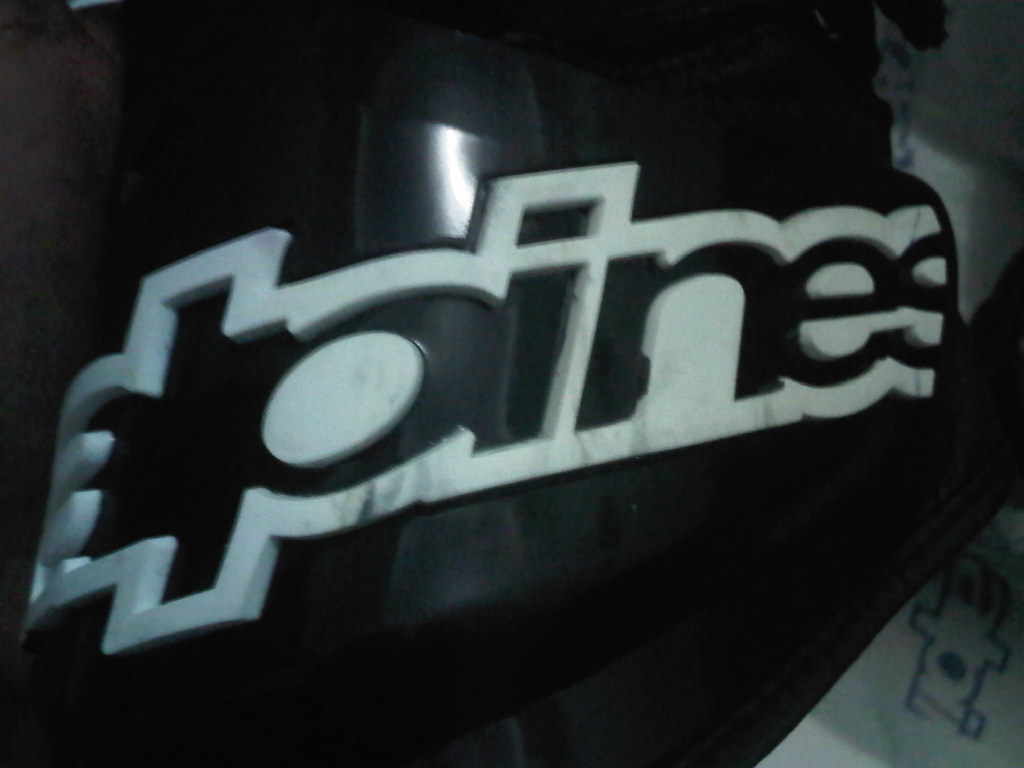The image is a large, square, predominantly black, white, and gray photograph taken from above. It features a slightly blurry, glossy black plastic object occupying most of the frame, possibly resembling a dome or the top of a helmet. This object notably has a 3D raised logo at its center with the word "pines" in bold lowercase black letters, outlined in white. The letter 'P' is distinctively highlighted with a white center. The black letters are embedded within a white, marble-effect embossed plastic structure.

In the lower right-hand corner of the image, there is a light gray surface with some sort of drawing on it in black, as well as a piece of paper with blue text that is partially visible. There is another section with a white plastic part and writing on it in the top right-hand corner. The image seems to have been taken in a dimly lit room, where the lighting highlights the shiny, reflective quality of the black plastic surface.